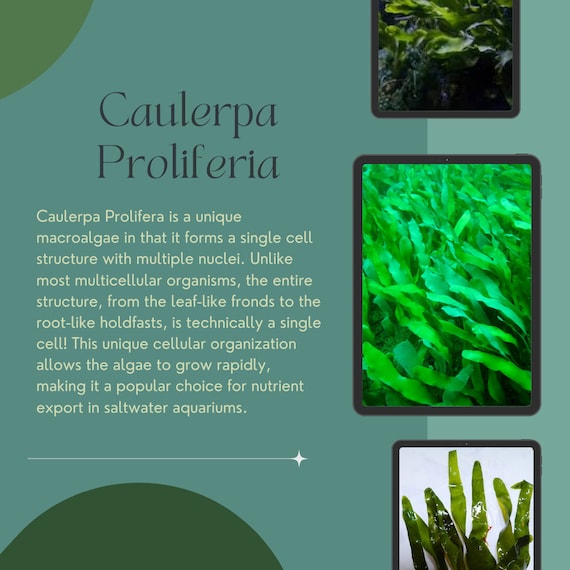The infographic features a plant called *Caulepa prolifera*, set against a dark green background. It includes a column of three distinct images with black frames on the right, showcasing different stages and parts of the plant. The main text, highlighted in light yellow, describes *Caulepa prolifera* as a unique macroalgae notable for its single-cell structure with multiple nuclei, encompassing both the leaf-like fronds and root-like holdfasts. The text details how this cellular organization supports rapid growth, making the algae a favored choice for nutrient export in saltwater aquariums. To emphasize the plant's subject, various shades of green are used, and there are decorative shapes enhancing the overall layout.